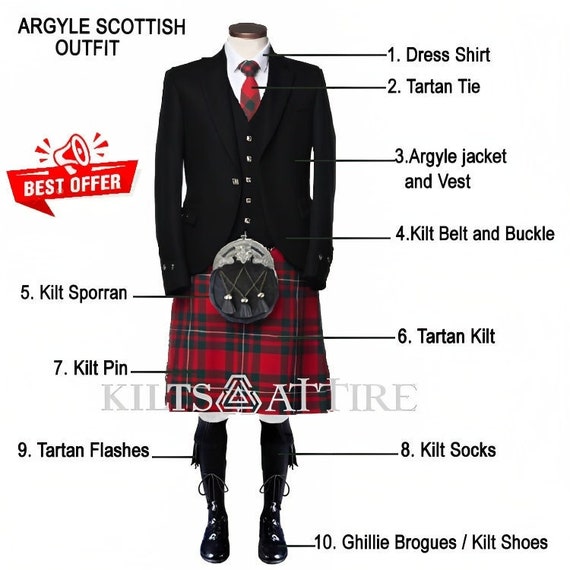This image features a headless mannequin dressed in a detailed Scottish Argyle outfit, primarily featuring colors of red, black, and white. Each element of the outfit is meticulously labeled and numbered from 1 to 10. The mannequin is adorned with a white dress shirt (1) topped with a red and green tartan tie (2). Over the shirt is a black vest and jacket ensemble, noted as the Argyle jacket and vest (3). The waist is cinched with a kilt belt and buckle (4), beneath which rests a traditional sporran (5). The centerpiece of the lower half is a tartan kilt (6), mirroring the tie's red, green, and white pattern. Complementing the kilt is a kilt pin (7), while knee-high black kilt socks (8) are further accentuated with tartan flashes (9). Completing the outfit are black ghillie brogues, or kilt shoes (10), featuring typical lace-up design with tassels. The text on the image suggests it could be a promotional diagram for a sales or rental listing by a company named "Kilt's Attire," offering the "Best Offer" for this ensemble.